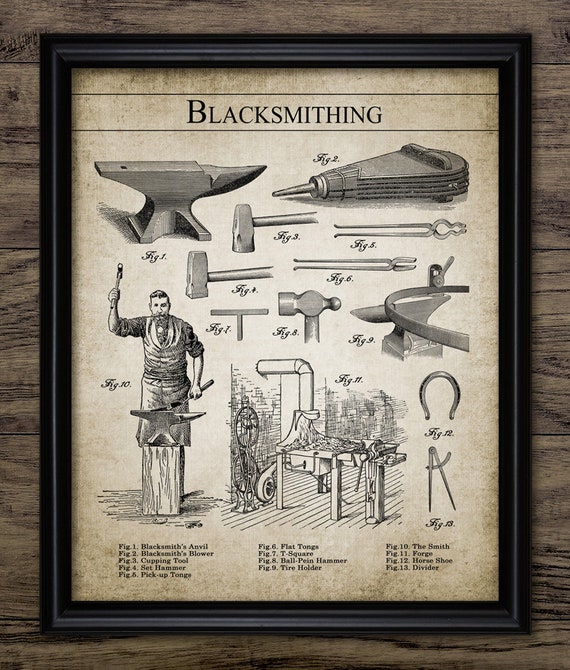The framed poster, encased in a thick black frame, is set against a background of light tannish wooden planks with significant dark graining, arranged horizontally. The poster itself exudes an old, vintage feel with a dirty gray hue accented by smears of dirt and wears a brown-beige tone. At the top, bold black lines frame the title “Blacksmithing,” beneath which an array of intricately drawn blacksmith tools is displayed in gray-scale illustrations, resembling a chart. 

Highlighted tools include an anvil and a bellows with a pointy tube, crucial for maintaining the fire. Three different types of hammers and several pairs of pliers are meticulously illustrated. Additionally, there is a depiction of chopstick-like rods. Below the tools, a detailed drawing of a blacksmith in action is shown. The man holds a mallet poised to strike an object on his maul, which rests on a sturdy tree stump. An explanatory section at the bottom of the poster reveals descriptions and uses for each depicted tool, providing a comprehensive overview of the blacksmith's craft.